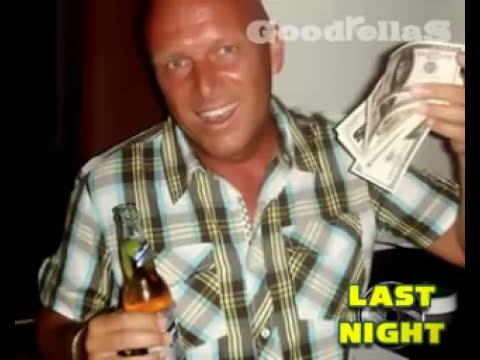The image features a clean-shaven, bald Caucasian man with slightly sunburned, tan skin and very light eyebrows, giving the impression of being almost non-existent. He is wearing a short-sleeved plaid shirt with a color pattern that consists of white, gray, light blue, pale yellow, green, and blue stripes.

The man seems to be in a festive or partying mood, evident from his tilted head and open-mouthed smile. In his left hand, he holds an open bottle of Corona beer with a lime inserted into it, suggesting he has either not drunk it or just started. His right hand proudly displays a few bills of undetermined currency.

In the image’s background, there’s a plain white area with a brown post visible behind him. Overlaying part of the image, in the upper-right corner, is the white transparent text "Goodfellas." Additionally, bright yellow text with a blue outline at the bottom corner reads, "Last Night,” reinforcing the revelrous theme of the picture.